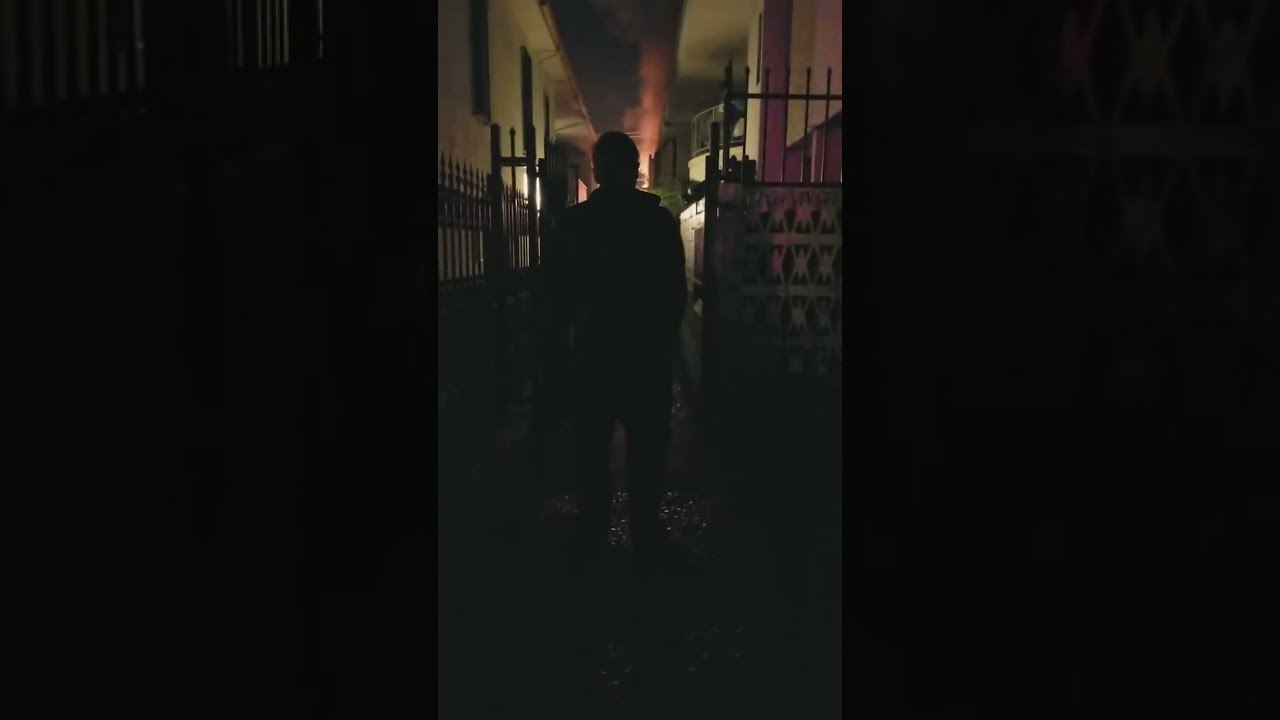The image is a very dark photograph, framed with large black bars on the left and right, creating a portrait orientation. In the center, a narrow alleyway stretches ahead, flanked by cream-colored buildings with a few windows and tall black wrought iron fences. The ground appears spattered with raindrops or water, adding texture to the shadowy scene. Prominently featured is the silhouette of a man, identifiable by his body shape and jacket, standing at an entrance through a wrought iron gate. The dimly lit setting is accentuated by a reddish glow behind him, giving the sky a misty or cloudy appearance. Despite the dark surroundings, there's a soft illumination that outlines his figure, enhancing the eerie ambiance of the nocturnal scene.